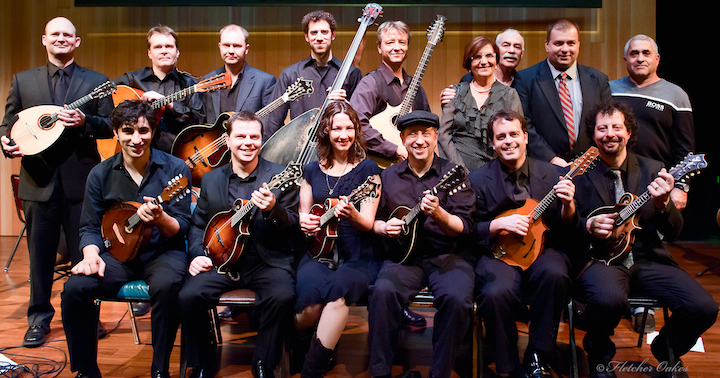This image is a professionally taken, rectangular photograph featuring a group of fifteen people organized into two rows, set against a backdrop of wood-paneled walls and a wooden floor. In the back row, nine individuals are standing, with the five men on the left holding various string instruments resembling a blend between guitars and violins. The remaining four people in the back row, consisting of three men and one woman, are not holding instruments. The men in the back row are dressed in dark suits, while the woman is wearing a dark gray ruffly shirt. In front of them, six people are seated on small chairs, including five men and one woman. Each of the seated individuals is holding a similar string instrument. The men in the front row are all clad in black dress shirts and pants, with some in full black suits, and the woman is dressed in a dark blue dress. All the members of the group are smiling, exuding an air of happiness and warmth, suggesting a recently ended performance or a celebratory occasion. The harmonious blend of their dark attire and joyous expressions creates a cohesive, cheerful atmosphere.